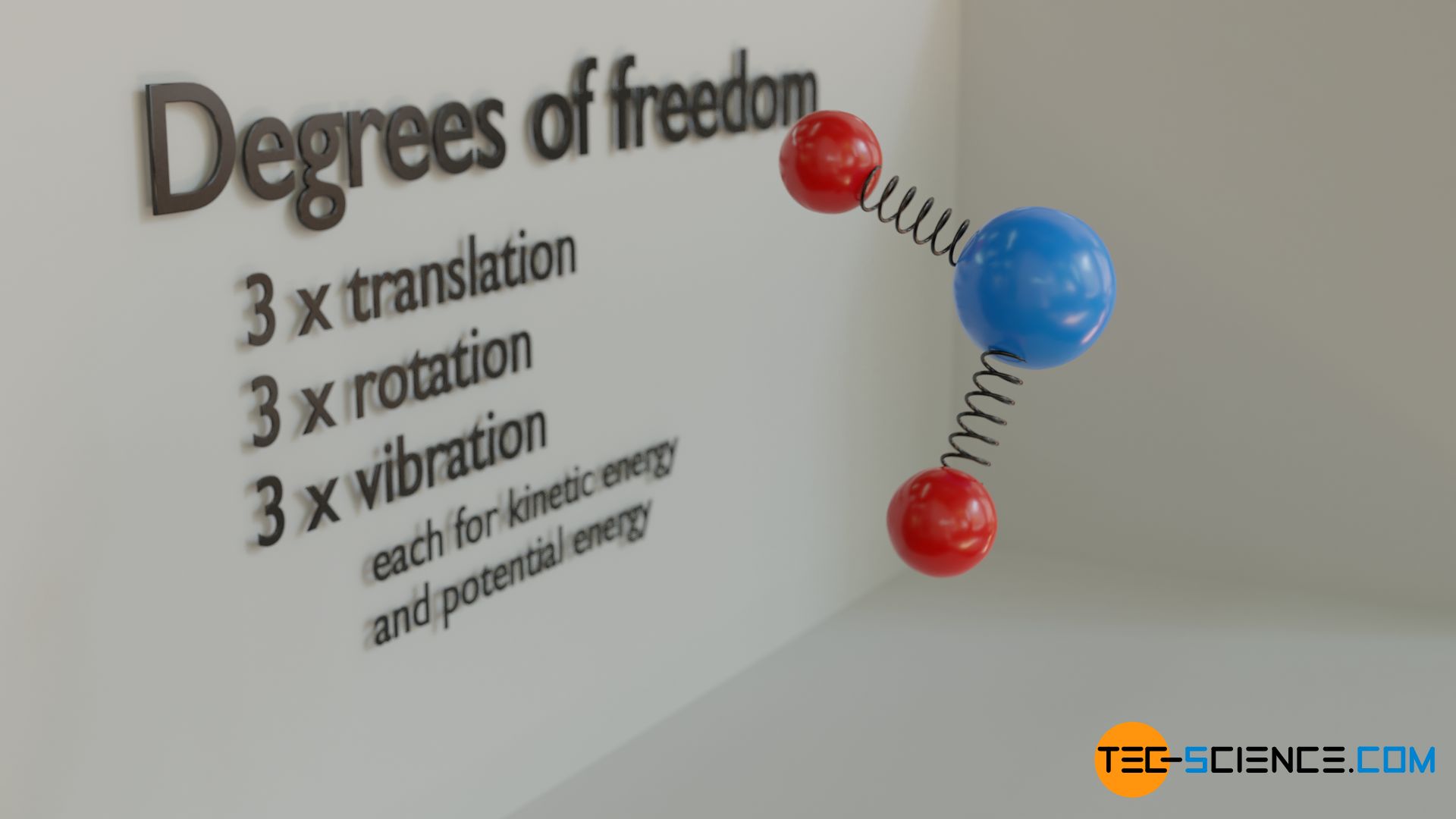This detailed caption describes the image accurately while cleaning up the spoken description for clarity:

"In the image, a well-crafted display prominently features a 3D atomic model. At the bottom of the photo, the TechScience.com logo is displayed in a stylized font, representing the company. The centerpiece of this display is a detailed atomic model: a central blue ball connected to two springs, each of which ends in a red ball, symbolizing atoms or molecules. 

To the left side of the photo, explanatory text breaks down the degrees of freedom for molecular motion. It states 'Degrees of Freedom' at the top, followed by '3x Translation,' '3x Rotation,' and '3x Vibration,' each on separate lines. Below this, in a smaller font, it clarifies that these degrees of freedom apply 'each for kinetic energy' and 'potential energy' on the final line. 

The text and the atomic model are mounted against a clean, white backdrop, possibly made of cardboard or foam core. Overall, the setup resembles an informative scientific display designed to educate viewers on molecular motion and energy states."